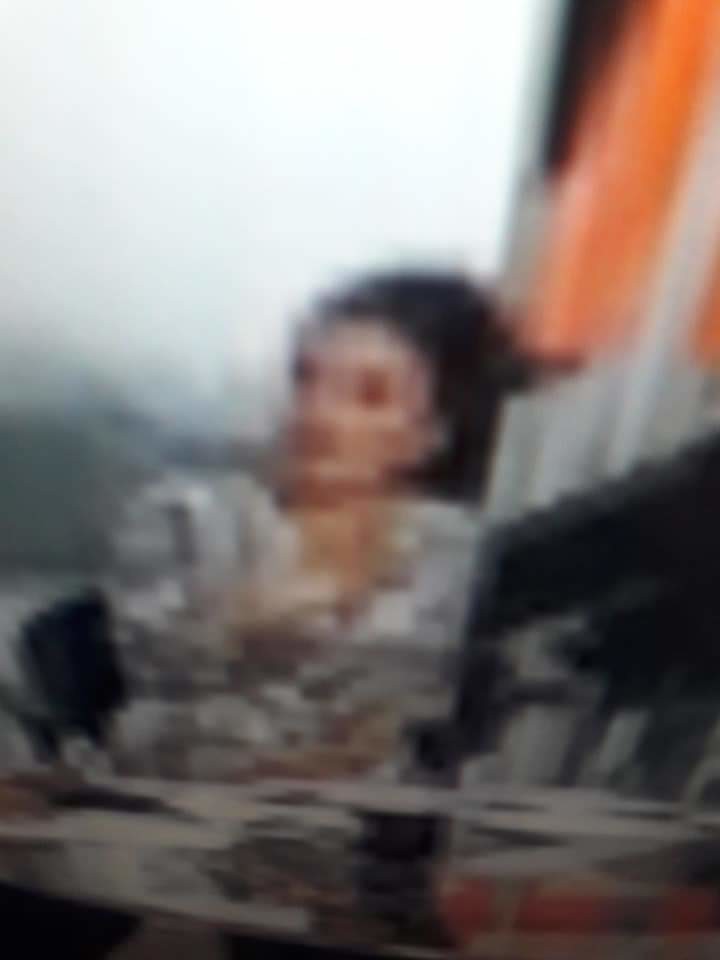The image is an exceptionally blurry photo, possibly reflecting a vintage style reminiscent of the 1950s. It prominently features a woman dressed in a mottled gray and white outfit with large shoulder pads or puffed sleeves. Her dark black hair is styled in an updo, possibly a bun or chignon. The woman is positioned towards the front, her face turned to the left of the image. A wisp of color, blending white and orange hues, envelops her shoulder, resembling smoke. The background is equally blurry and predominantly white, with a feature in the upper right that could be a flag or banner showcasing orange and white colors. The overall impression combines elements of a nostalgic scene with unclear contextual details, suggesting a moment captured from an old, colorized photograph.